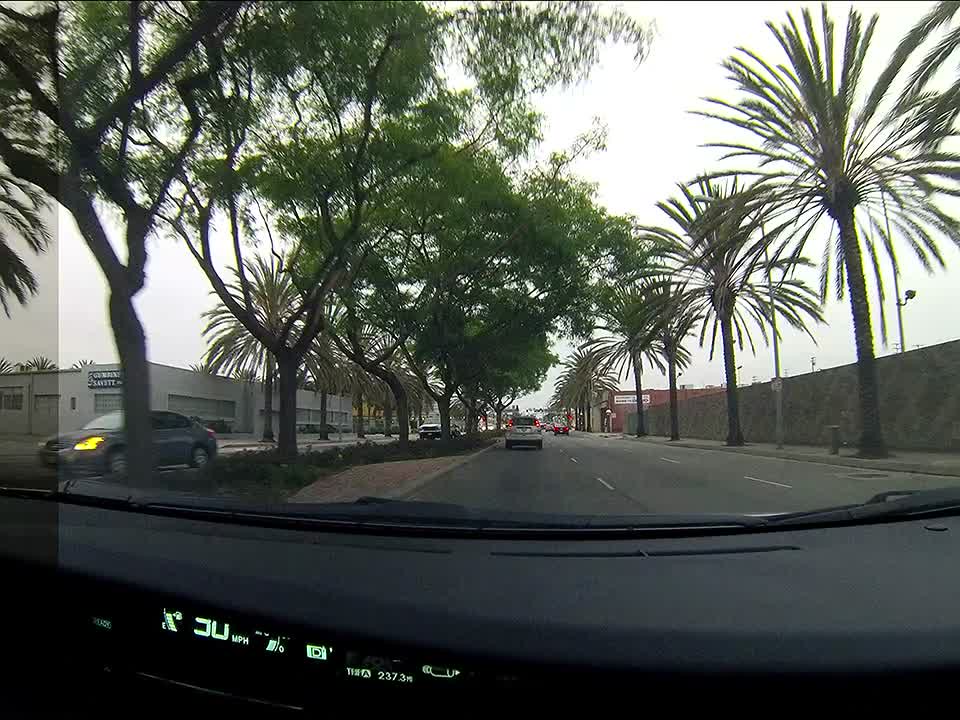A view through a car windshield captures a multi-lane road scene. The car's black dashboard is partially visible, along with a fragment of the digital display on the lower left. Positioned in the far left lane, the car navigates a three-lane street with a central median lined with trees. Adjacent to the center divider, opposite lanes accommodate oncoming traffic. A gray sedan is seen towards the left, behind which stands a two-story gray business building. Directly ahead, a gray SUV with illuminated brake lights can be seen. In the adjacent lane, a red car waits at a traffic light. To the right, a series of palm trees line the street, bordered by a brown fence. The day is bright and clear, accentuating the orderly arrangement of the scene.